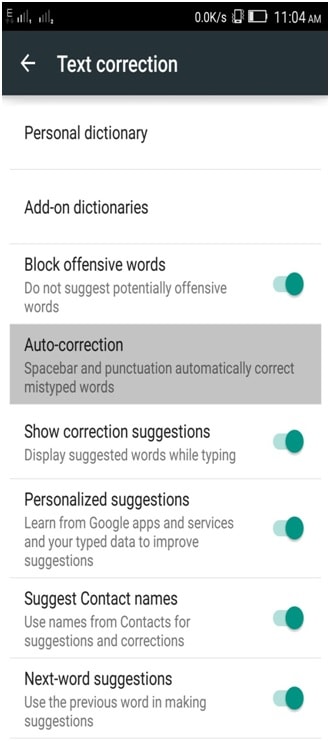This image shows a smartphone screen displaying its text correction settings menu. 

At the top of the screen, the status bar indicates a few details: an 'E' symbol suggesting emergency services, a signal strength icon with two bars, and a data transfer rate of 0.0 K/s. Additionally, there is a phone icon indicating the device is set to vibrate, a low battery icon, and the current time displayed as 11:04 AM.

Below the status bar, the screen displays the text correction settings menu with several options available for selection:
1. **Personal Dictionary**
2. **Add-on Dictionaries**
3. **Block Offensive Words:** This option, which prevents suggestions of potentially offensive words, is activated as indicated by the switch being set to 'on'.

Following these options, enclosed within a dark gray box, is:
- **Auto Correction:** Described as automatically correcting mistyped words using the space bar and punctuation.

Below this box, there are four more toggles, all of which are currently turned on:
1. **Show Correction Suggestions:** Displays suggested words while typing.
2. **Personalized Suggestions:** Learns from Google apps and services as well as your typing data to improve suggestions.
3. **Suggest Contact Names:** Uses names from contacts for suggestions and corrections.
4. **Next Word Suggestions:** Utilizes the previous word to make better suggestions.

Overall, this detailed screenshot captures various text correction features and settings currently activated on the smartphone.